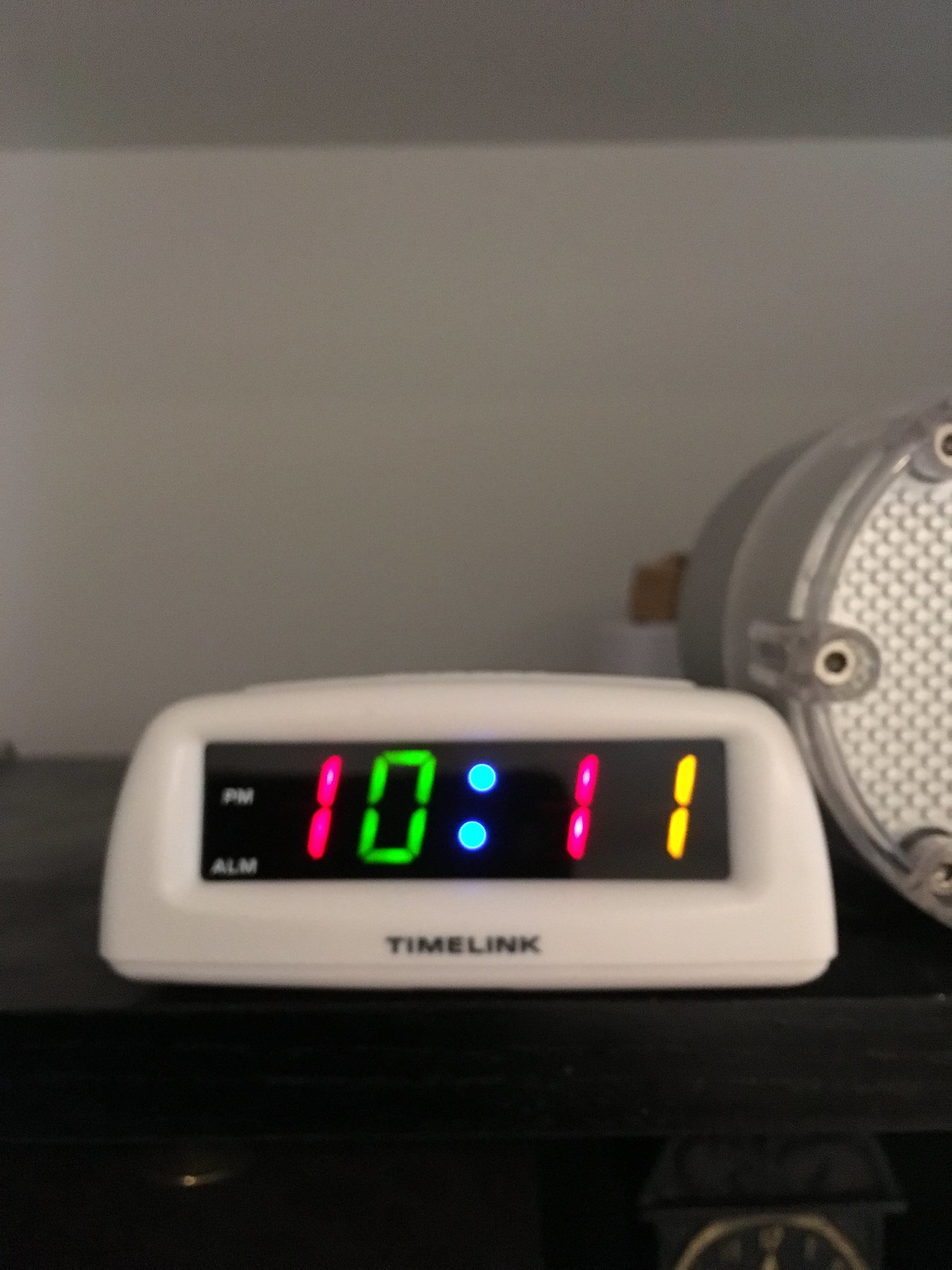This image showcases a Timelink alarm clock with a white rectangular body and a black face. The clock displays digits in vibrant neon colors: the first number '1' is neon pink, '0' is neon green, and the two separating dots glow in neon blue. The second '1' is neon pink, while the final digit is an eye-catching neon orange-yellow. Above the display, there are small labels indicating "FM" and "Alarm." The clock is positioned on a black night table, beside a lamp that resembles a spotlight. Underneath the table, a black object with copper accents is partially visible.